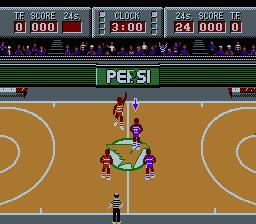In this detailed square image, the screen showcases a video game simulating a basketball match. The court stretches horizontally in a pale orange hue. Four digitally-rendered players occupy the court: two wearing blue and white uniforms positioned on the right and two in red and white uniforms on the left. Above the court, an array of digital spectators is visible, represented by mere outlines of heads and upper bodies. Spanning the top of the image is a broad gray scoreboard. On the left upper corner, the scoreboard reads "0, 0, 0." Centrally placed, the word "CLOCK" appears, with "3 o'clock" displayed directly beneath it. To the right is "24," likely indicating a 24-second shot clock. Both scores display "0," and the abbreviation "TF" also shows "0."